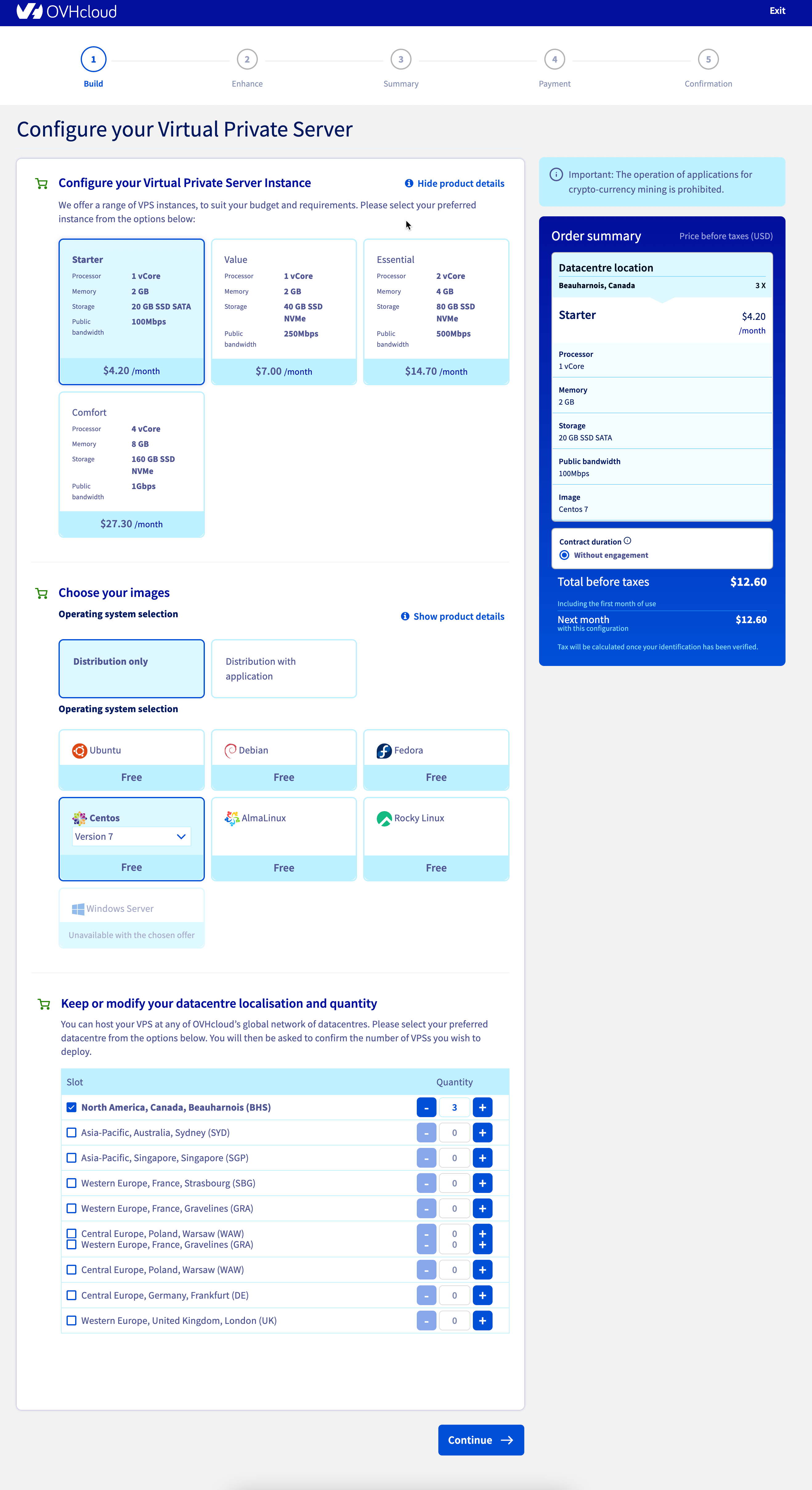The image depicts the first step in configuring a Virtual Private Server (VPS) through a user interface. At the top of the page, a timeline status bar outlines the five steps of the process: Build, Enhance, Summary, Payment, and Confirmation, with the current focus on the Build step. 

The page's content is densely packed, featuring small text that can be challenging to read. The build page invites users to configure their VPS instance by selecting various options. 

Initially, users can choose from four VPS tiers, with the default selection being the "Starter" tier, priced at $4.20 per month. While the specific features of each tier are listed, they are not easily readable. Further down, users are prompted to select their preferred operating system, with options including both Windows and an array of Linux distributions.

Additionally, the page offers the option to retain or modify data center localization and quantity. A list of data center locations is provided, with North America selected by default.

This detailed description highlights the core aspects and user options available on the VPS configuration page.